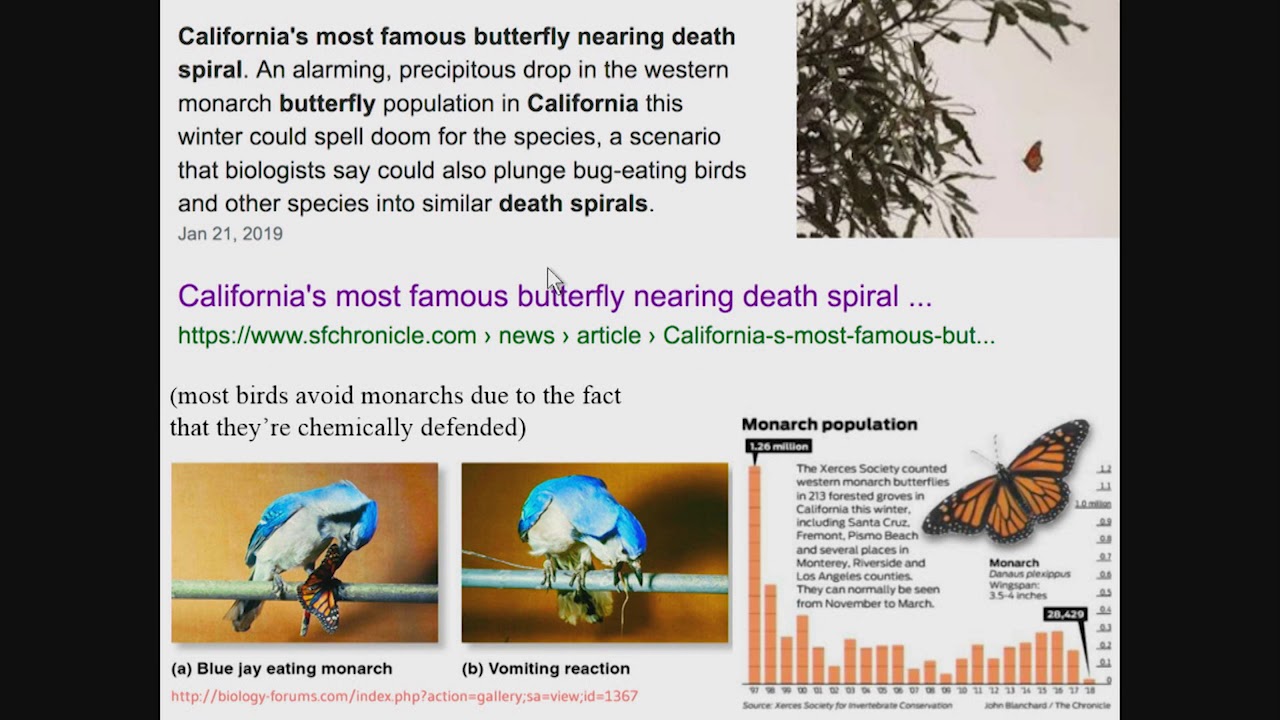**In-Depth Caption:**

The screenshot features an alarming report concerning the drastic decline of the western monarch butterfly population in California. Set against a black background, the main headline boldly states, "California's Most Famous Butterfly Nearing Death Spiral." This highlights the significant drop in the monarch population during the winter of January 21, 2019, which threatens the butterfly species with potential extinction. The text warns that this decline could trigger similar downward trends for bug-eating birds and other species, emphasizing the ecological impact.

Visual elements in the screenshot include two pictures labeled with the letter "A." The first image captures a blue jay consuming a monarch butterfly. The second image displays the bird with its mouth open, accompanied by text indicating a vomiting reaction due to the monarch's chemical defenses. A red link and a gray square with the label "Monarch Population" also appear, featuring an additional image of the butterfly.

Overall, the detailed report underscores the urgency of the situation, depicting both the monarch's plight and its broader implications on the ecosystem.